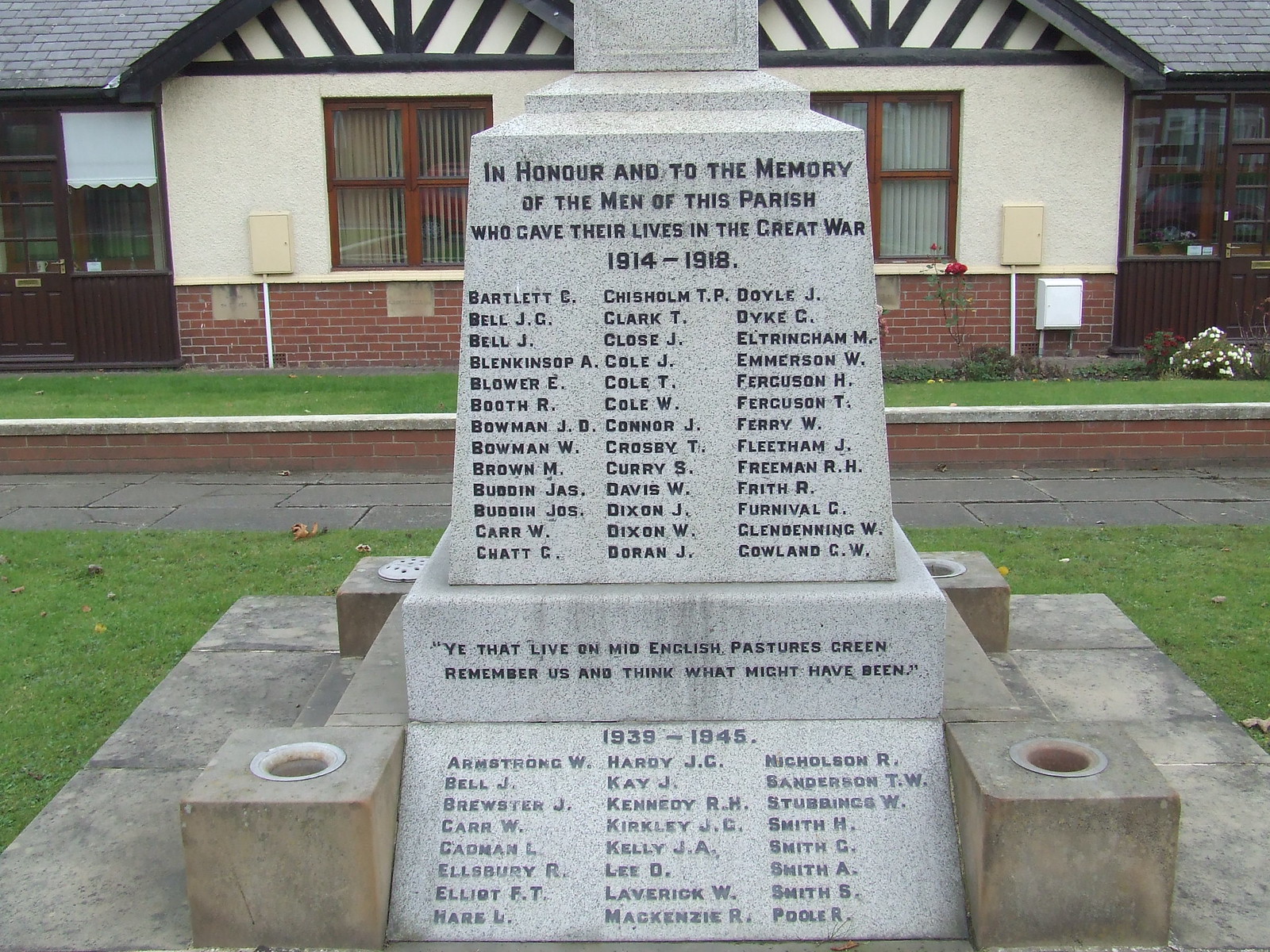This color photograph captures a somber outdoor scene featuring a large, square-shaped stone memorial dedicated to the men of a parish who gave their lives in the Great War of 1914-1918 and World War II from 1939-1945. The monument, positioned on a substantial gray stone platform and flanked at each corner by square stone bases with decorative holes, stands prominently in front of a one-story building with stucco siding and brick lower walls. The building also features wooden frame glass windows and a low brick wall in the foreground.

The side of the memorial facing the camera bears the inscription: "In honor and to the memory of the men of this parish who gave their lives in the Great War 1914 to 1918." Below this, the names are listed alphabetically from Bartlett to Gowland, including, but not limited to, Bartlett C, Bell J C, Bell J, Blenkinsop A, Blower E, Booth R, Bowman J D, Bowman W, Brown M, Clark T, Close J, and Cole J. Further down, a poignant quote reads: "Ye that live on Mid-English Pastures Green, remember us and think what might have been." Beneath this, the dates "1939 to 1945" appear, followed by another list of names starting with Armstrong W and ending with Pooler.